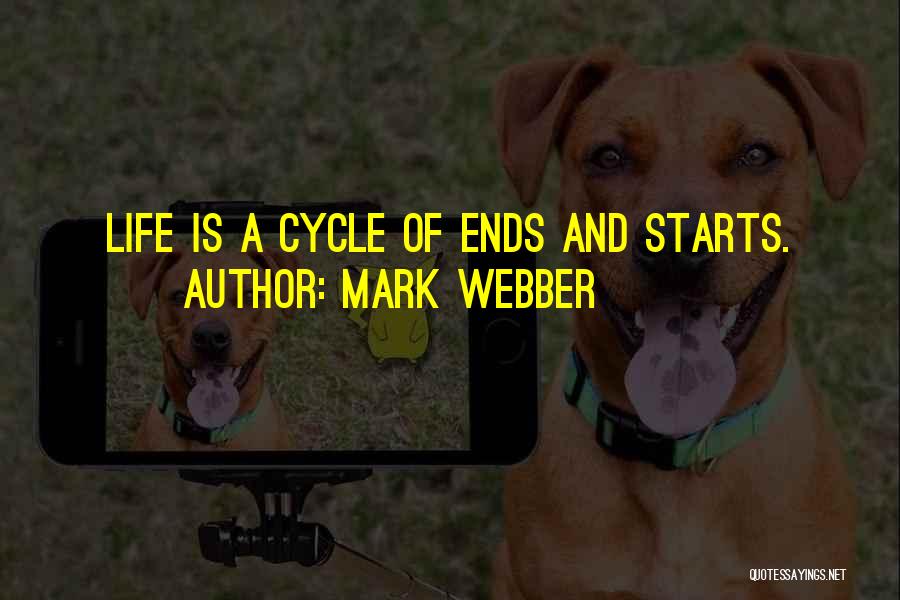The image features a light brown dog with floppy ears and a speckled black-dotted tongue, sitting on a grassy field and looking directly at the camera. The dog, which seems to be a pitbull mix wearing a green collar, is the primary focus. Captured on a smartphone held on a selfie stick, the phone’s screen shows the same dog along with a cartoon Pikachu on the right side. The entire image has a black tint and is overlaid with yellow text that reads, "Life is a Circle of Ends and Starts," attributed to author Mark Webber. The watermark "quotesayings.net" is discreetly positioned in the bottom right corner.